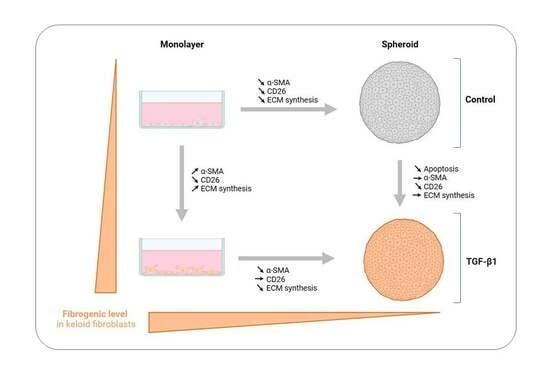The image features a detailed educational diagram on a white background. At the top, there are labels for "Monolayer" on the left and "Spheroid" on the right. Beneath the "Monolayer" label, there is a pink and white rectangle, predominantly pink. Below this rectangle, an arrow points towards additional text annotated with several terms, such as alpha-SMA, CD26, and ECM synthesis. 

Further down, there is another pink and white container featuring an orange triangle on the left, labeled "Fibrogenic level in keloid fibroblasts." An orange arrow extends from this triangle to the right. There are several other arrows and shapes within the diagram, including circles and more arrows pointing in various directions, indicating complex interactions and processes.

To the right, near the "Spheroid" label, there is a gray circle with a beehive pattern inside it. Further details include labels for "Control," "TGF beta 1," and other annotations such as apoptosis, alpha-SMA, CD26, and ECM synthesis, which are linked by arrows suggesting a flow of information or process. The entire content is enclosed within a gray rectangular border that organizes these components into a cohesive visual explanation.